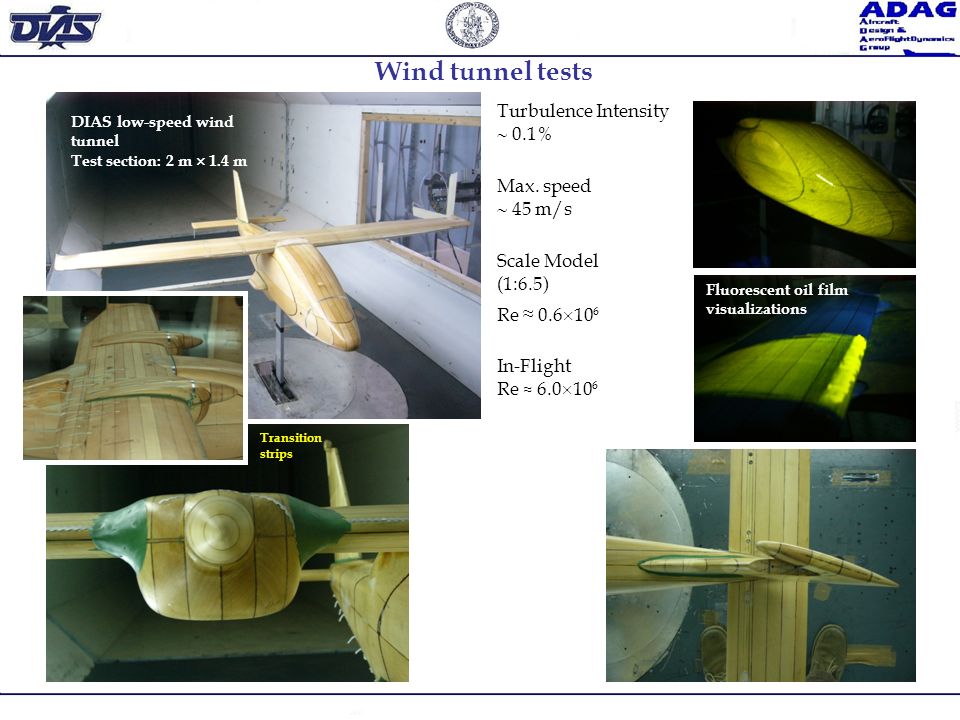The slide from the PowerPoint projection appears to be a detailed overview of wind tunnel tests conducted on model airplanes by the Aircraft Design and Aerodynamics Group (ADAG). In the upper left corner, there is an emblem with an eagle and the acronym D-I-A-S. The central part of the slide features a circular crest logo and bears the title "Wind Tunnel Tests." On the upper right, the text identifies ADAG along with the full name "Aircraft Design and Aerial Flight Dynamics Group."

The slide showcases six pictures of what seems to be different models of wooden airplanes in a wind tunnel. The upper left image displays a wooden airplane labeled "D-I-A-S, Low Speed Wind Tunnel, Test Section 2 meters by 1.4 meters." The next image below is a close-up of a wooden airplane wing, while the bottom left image highlights transition strips with yellow text. 

On the right side of the slide, the top right picture shows a model with a glowing yellow piece against a blue background, followed by another image labeled "Fluorescent Oil Film Visualization," illustrating a similar yellow piece. The final picture on the bottom right appears to be a partly drawn scene, showing feet standing on a wooden board over a blue backdrop.

The central part of the white background between the images includes data such as turbulence intensity approximately 0.1%, maximum speed around 45 meters per second, a scale model ratio of 1:6.5, Reynolds number (RE) approximately 0.6 x 10^6, and in-flight RE roughly 6.0 x 10^6. 

The model airplanes are predominantly light brown with some green embellishments on one of the planes, suggesting different variations and details observed during the tests. A horizontal black line runs at the bottom underneath the pictures, finalizing the layout.